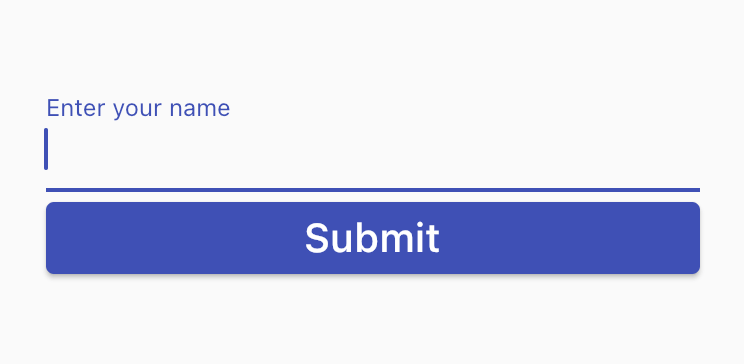A close-up of the bottom portion of a mobile phone screen displays a minimalist user interface. The white background enhances the simplicity of the layout, which features two primary elements: an input field and a submit button. Centered towards the top is a prompt in blue text that reads, "Enter your name." The text is rendered in a smaller font size, likely 12pt, with only the first word capitalized. Directly below this prompt is a blue line suggesting where users should input their name, accompanied by a blinking cursor.

Prominently placed below the input field is a large, rectangular blue button inscribed with the word "SUBMIT" in uppercase white letters, estimated to be in an 18pt font. The interface design relies exclusively on the colors blue and white, ensuring a clear and straightforward user experience. The overall image is uncomplicated, focusing solely on these essential components, indicative of a user being prompted to enter their name and submit it through the app.